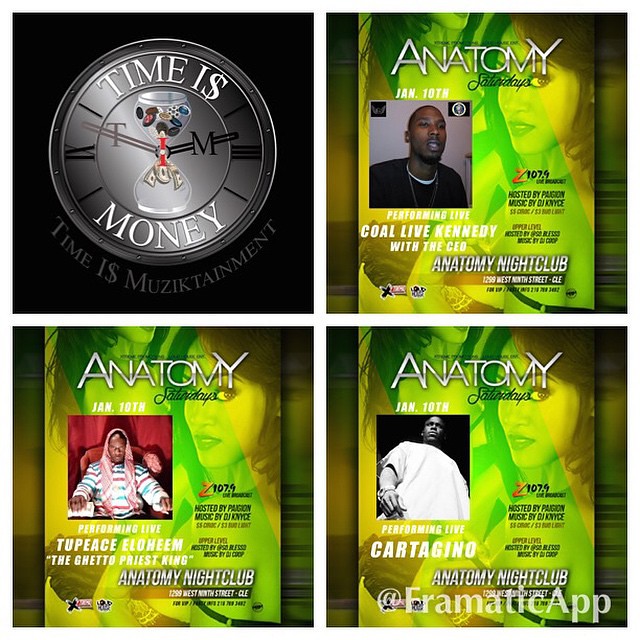The image is divided into four quadrants, each representing a different aspect of a promotional campaign for "Anatomy Saturdays." The top-left quadrant features a logo against a black background, depicting a silver clock with the phrase "Time is Money" encircling it. The 'S' in 'is' is stylized as a dollar sign, and instead of sand, the hourglass dispenses money. Small clock faces are visible within the hourglass, symbolizing the fusion of time and wealth. Below the clock, it reads "Time is Music Attainment" in gray font.

The remaining three quadrants contain identical posters promoting an event at Anatomy Nightclub, located at 1299 West 9th Street, Cleveland. These posters are green with yellow accents and feature an attractive dark-skinned woman with arched eyebrows, looking over her shoulder in the background. Each poster also showcases a different performing artist. 

The top-right poster highlights Co-Live Kennedy, depicted in a black shirt with the title "Performing Live" beside his name. The bottom-left poster features Two-Piece Elohim, the Ghetto Priest King, distinguished by his striped shirt and untied do-rag while sitting in a chair. The bottom-right poster promotes Cartangeno, who is wearing a white shirt and is photographed from a low angle against a black background. Each poster includes a watermark with the Instagram handle, "Phramatic App."